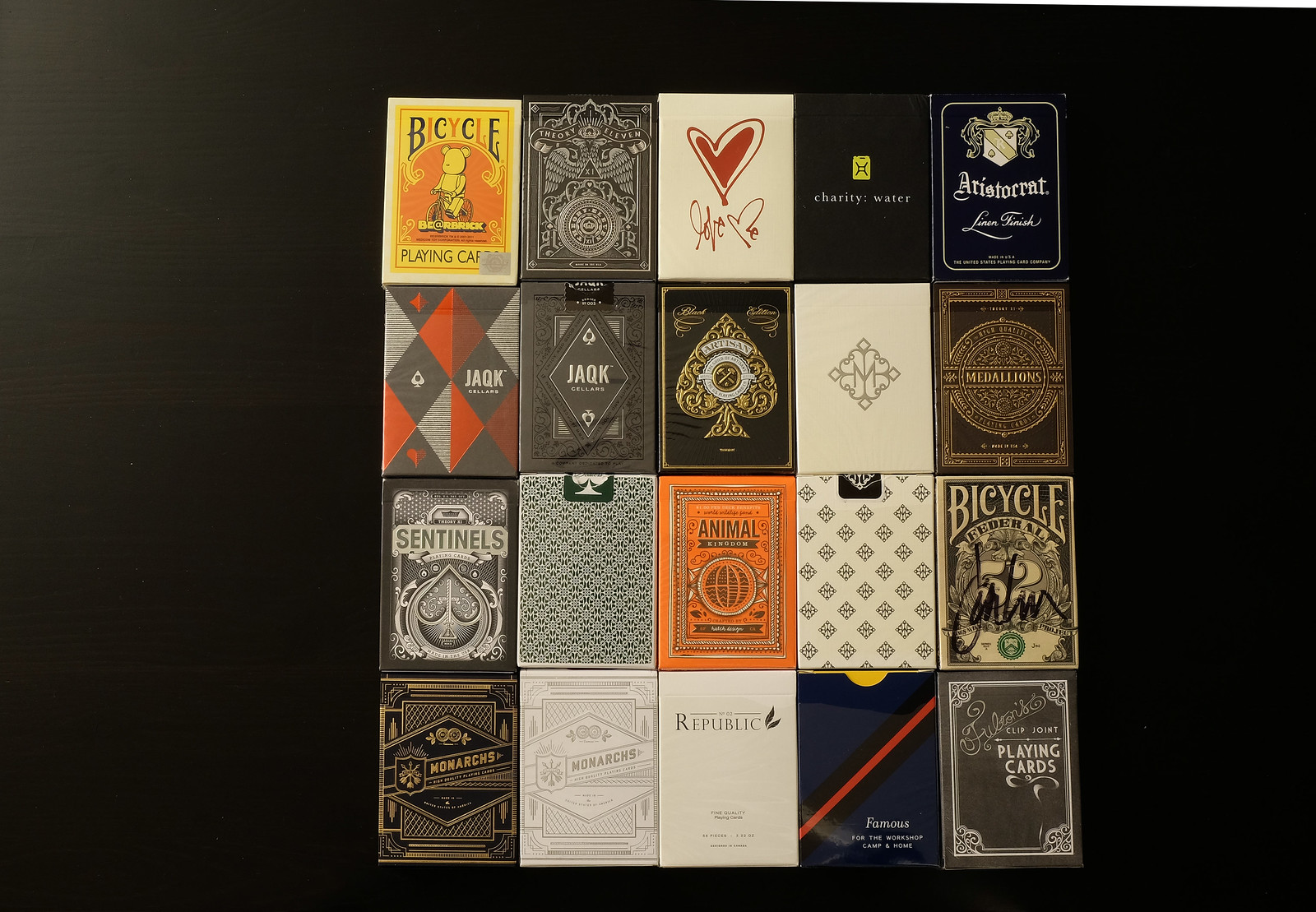This meticulously arranged photograph showcases 20 distinct packs of playing cards, each boasting unique and artistic designs. The varied color palettes and company logos lend an eclectic and visually engaging appearance to the collection, which is neatly set against a dark gray background, organized from left to right and top to bottom.

Starting in the top row, there's a vibrant orange and yellow pack from Bicycle, featuring a teddy bear riding a bike. Adjacent to it is a pack displaying a medallion with eagle wings, though the branding is hard to decipher. Next, a sleek white pack stands out with a modern design and what appears to be an autograph reading "Hefe Mi." Beside it, another pack features a small yellow logo with "Charity Water" inscribed in white letters. The row concludes with a navy blue pack embossed with a white crest and the words "Aristocrat Linen Finish."

In the second row, a pack with orange and gray triangles bears the brand name JACCQ. A similar pack from the same brand follows, this time with a gray background and diamond logo. Next, a gray pack adorned with a gold filigree club shape seems to read either "Artesian" or "Aristocrat." Another pack, minimalistic in design, has a white background with the letter "M" and a simple crest. Completing this row is a taupe-colored pack featuring an intricate medallion design and the word "Medallions" at its center.

The third row begins with a pack labeled "Sentinels," showcasing a gray background with a crest resembling some fruit. Following this is a plain pack with a comprehensive gray and white pattern, featuring a club shape on its label. An orange pack comes next, displaying a square inset design and a circle medallion labeled "Animal." Adjacent to it is a white pack decorated with diamond shapes that incorporate the letter "M." This row ends with a retro-looking Bicycle pack branded "Federal 52," with a signature resembling the name "Carlson."

In the final row at the bottom left, a gray and gold deck marked "Monarchs" features an ornate crest at the top and side. Next to it, a nearly identical design appears on a white background. A clean, white deck with the word "Republic" flanked by two gray leaves follows. The subsequent pack, by "Famous," presents a diagonal red line bordered with black and a small yellow label at the top. Concluding the collection is a gray pack labeled "Clip Joint Playing Cards," bearing an unreadable script.

This curated assembly of playing cards, diverse in both color and design, demonstrates the artistic individuality of each pack and the brands they represent.